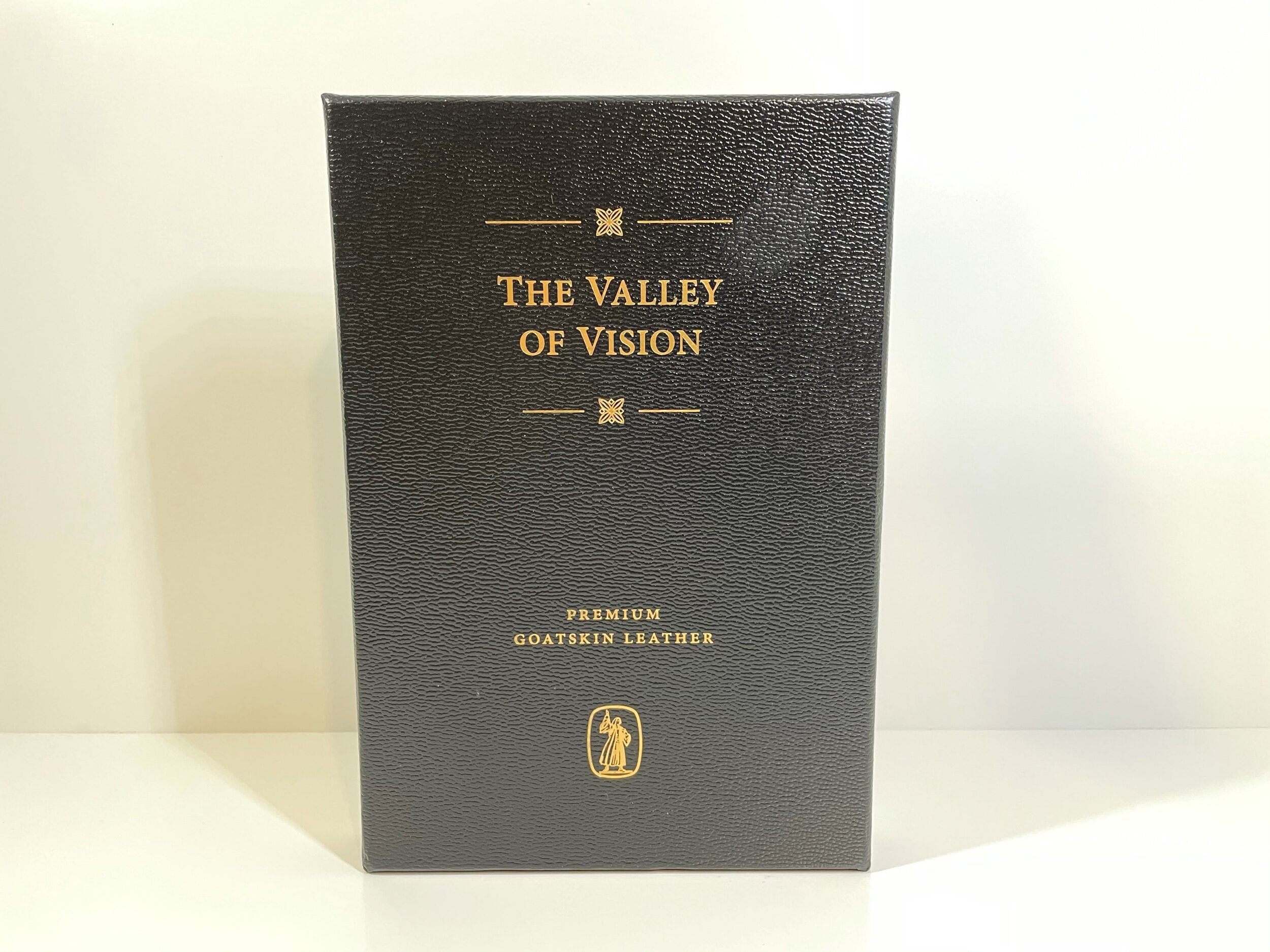The image features a black, rectangular item that could be a book, journal, or wallet, made of textured, premium goatskin leather. It is positioned on a plain white table with a white wall in the background. The cover showcases gold text and logos. At the top, "The Valley of Vision" is inscribed in gold between two intricate, gold-stamped lines. Below the title, the cover also bears the same two-line design with a small star-like figure in the center. Further down, "Premium Goat Skin Leather" is stamped in gold. At the bottom, there is a small, gold-outlined, rectangular icon depicting a person in a long robe, holding an arm upwards. The entire design, including all lettering and symbols, is rendered in gold on the textured leather cover.